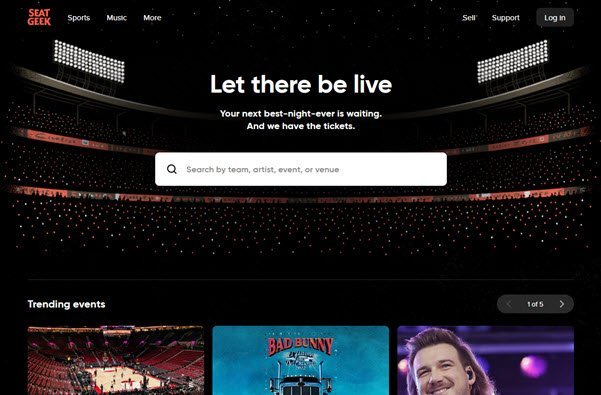In this horizontally elongated image, we see a photograph of a large stadium that is enveloped in darkness, save for the numerous small lights emanating from either lighters or cell phones held by attendees. This scattering of lights creates an enchanting effect, reminiscent of a starry night sky. Dominating the center of the image is a white search box with the placeholder text in light gray, "search by team, artist, event or venue." Above this search box, in large bold white text, is a captivating message: "Let there be live. Your next best night ever is waiting and we have the tickets." In the upper left corner, the brand "SeatGeek" is displayed in red text, and to the right of that are the categories "Sports," "Music," and "More." The top right corner of the image features options for "Support" and "Login." At the bottom of the image, three smaller thumbnail photos appear under the label "Trending Events." This meticulous and comprehensive layout entices viewers to dive into a world of live events and entertainment.